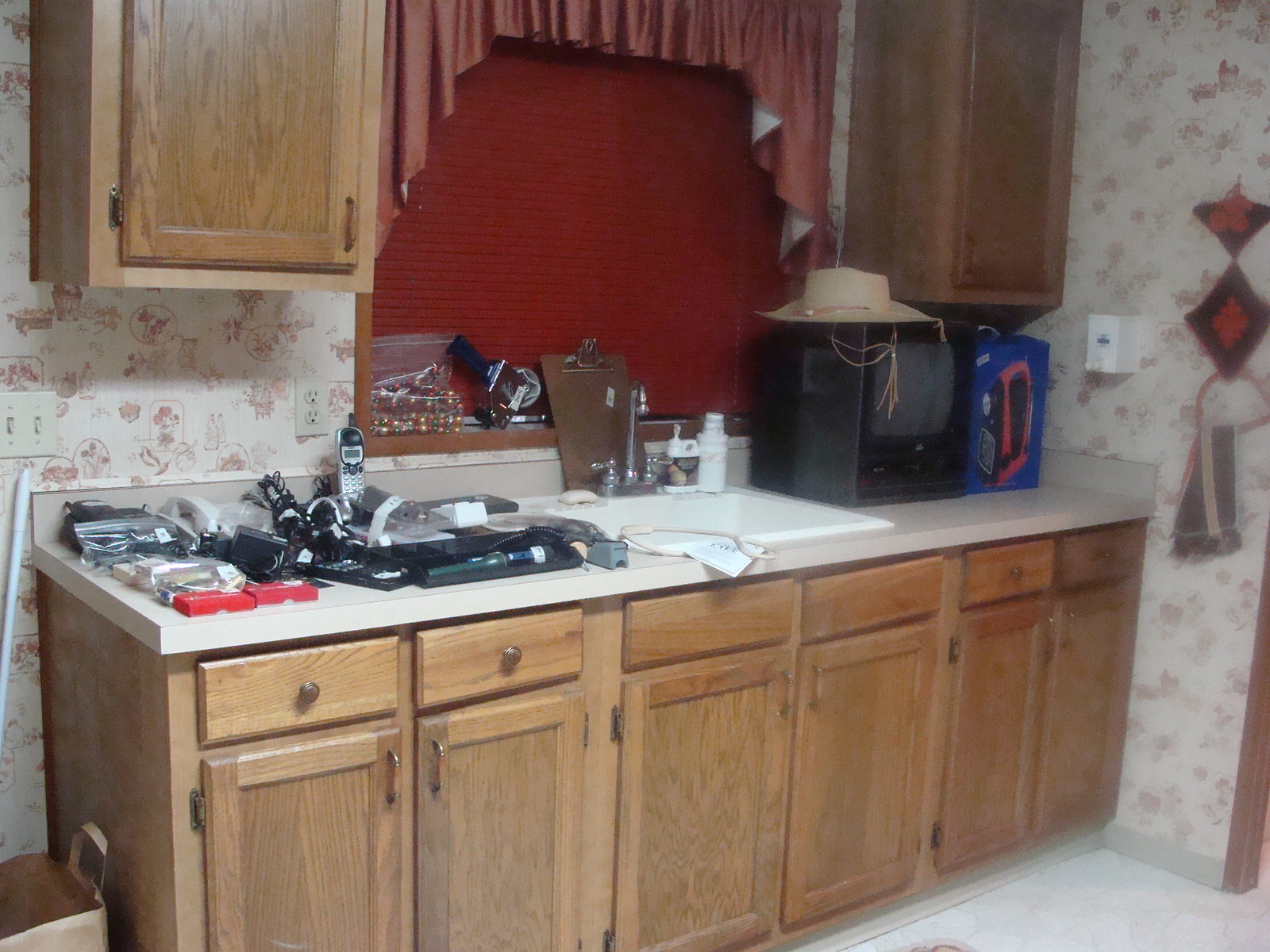The photograph depicts a well-used kitchen area with a central focus on the sink and surrounding countertops. The kitchen sink, prominently placed in the middle, is a classic white porcelain basin. Above it, a tall, chrome-plated spigot extends upwards, flanked by handles on both sides to control hot and cold water. 

To the right of the sink, the clean white countertop hosts an old 13-inch TV encased in black plastic. Adjacent to the TV, there is a box containing an emergency lighting and radio system, identifiable by its red handle and the combination of a light and radio embedded within it.

In contrast, the left side of the countertop is cluttered with various items, including a cordless phone, a flashlight, and several boxes with red tops that resemble checkbook boxes. This area appears more disorganized with numerous small items scattered across the surface.

Below the countertop, the kitchen cabinets are neatly arranged. There are four drawers, each fitted with a handle, as well as six pull-open cabinet doors, also equipped with handles. 

The window behind the sink is covered by a red shade, fully drawn down, obstructing the outside view. Flanking the window, there are additional cabinets on either side, integrated into the wall, providing both symmetry and extra storage space.